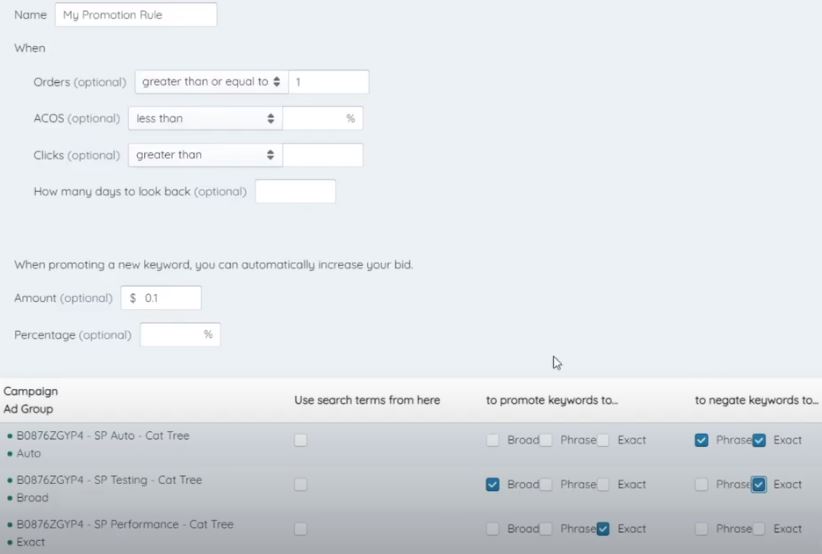Detailed Description:

This screenshot represents a section of a website where users can set various parameters for promoting and managing their keyword campaigns. The section starts with fields such as "Name" and "My Promotion Rule" followed by "When". Users can specify orders (with "Optional" indicated in parentheses), where values can be adjusted with up and down arrows. There is a box for "ACOS" (Advertising Cost of Sale), marked optional, set to accept a percentage value, indicated by a percentage sign within the box.

Next is the "Clicks" field, which is also optional, with the option to specify "greater than". There's also a field for "How many days to look back," again, marked as optional. Further down, there's an advanced option for promoting a new keyword where users can automatically increase their bid. The "Amount" field here is optional and currently displays "ten cents", not "one cent" as initially thought. There's also an "optional percentage" field left blank.

Underneath these settings, there's a section labeled "Campaign Ad Group", which includes options to use search terms from specified campaigns to either promote or negate keywords. Each function corresponds to an option in the top bar.

Finally, a list of campaigns is shown, each with unique identifiers, including "SP Auto", "CATTRI Auto", "SP Testing CATTRI Broad", and "SP Performance CATTRI Exact". These campaigns help in managing the performance and testing of different keyword promotion strategies.